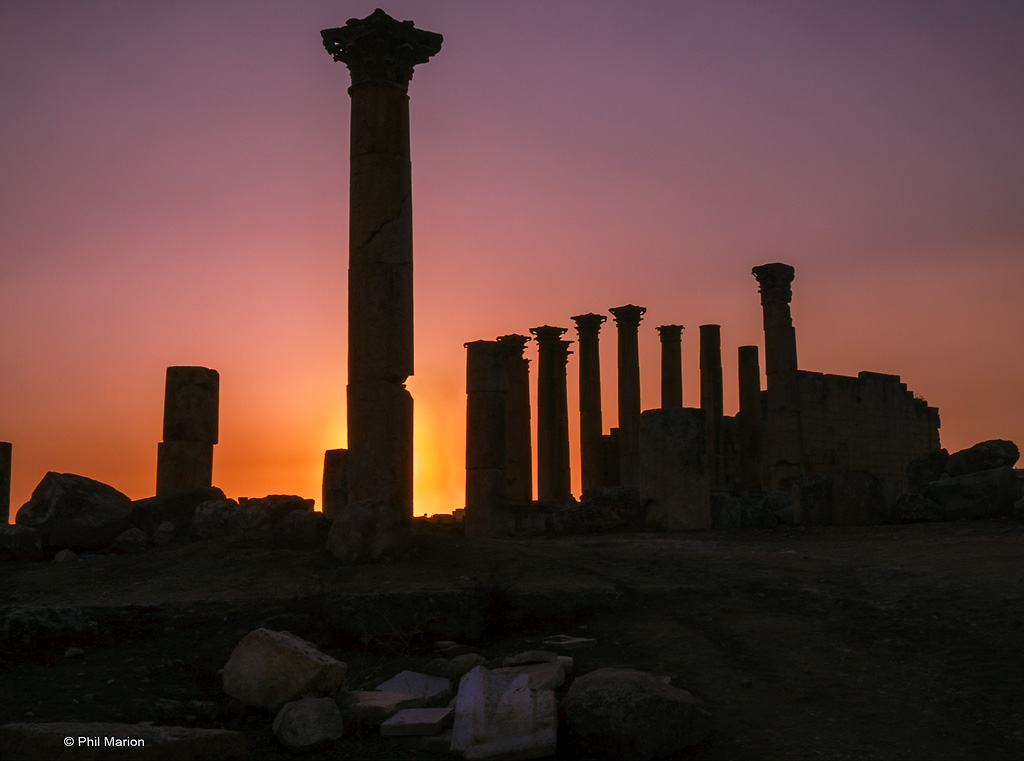This color photograph captures the evocative scene of an ancient ruin at sunrise or sunset, depicting a landscape steeped in history. Dominating the foreground are piles of crumbled rocks, the remnants of what was once a grand structure. Rising majestically into the sky, slightly left of center, is the tallest of the ten silhouetted columns, impressive and seemingly precarious with a noticeable crack near its base and additional cracks fanning out at the top. To the right, a series of shorter columns lead the eye toward a mostly crumbled wall that remains partially intact. The dramatic sky enhances the historic ambiance, transitioning from a glowing yellow near the horizon, through shades of orange and pink, and culminating in a deep purple overhead. The largest column stands directly against the backdrop of the glowing sun, creating a striking silhouette in dark contrast to the colorful sky. In the bottom left-hand corner, the photographer’s name, Phil Marion, along with a copyright symbol, is subtly inscribed in white text, adding a professional watermark to this captivating and serene scene.